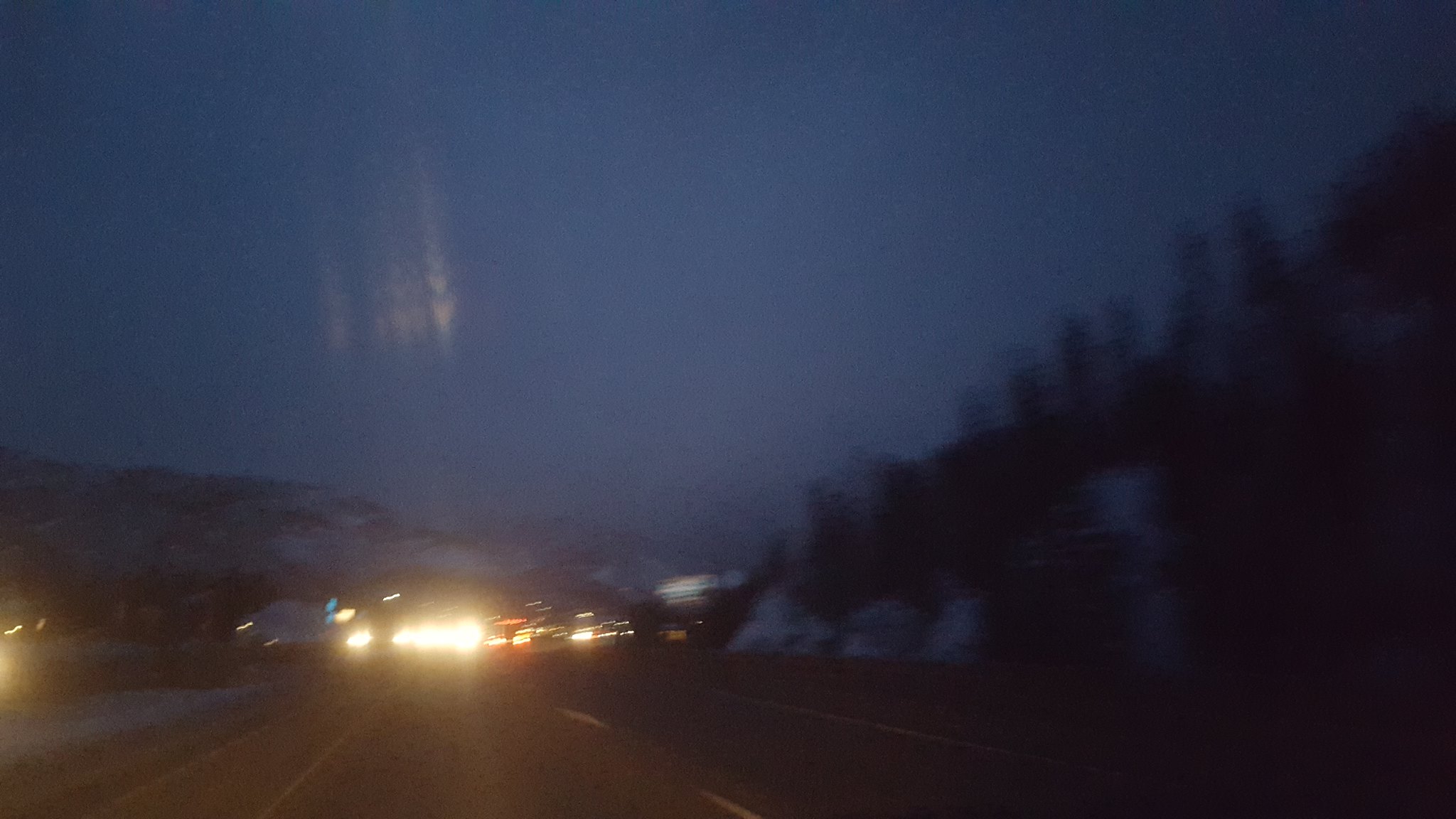A landscape-oriented photograph captures a nighttime scene from a road perspective. The image is noticeably blurry, suggesting it was taken from a moving vehicle. The time appears to be late dusk, as the sky is a dark blue but still slightly illuminated, and it looks overcast. The headlights of oncoming traffic on what appears to be the opposite lane—on the left side of the image—create noticeable glares. The yellow lines marking the lanes are faintly visible at the bottom of the frame. On the right side, there is a vague outline of trees or some form of roadside landscape, but the blurriness makes it difficult to definitively identify these features.